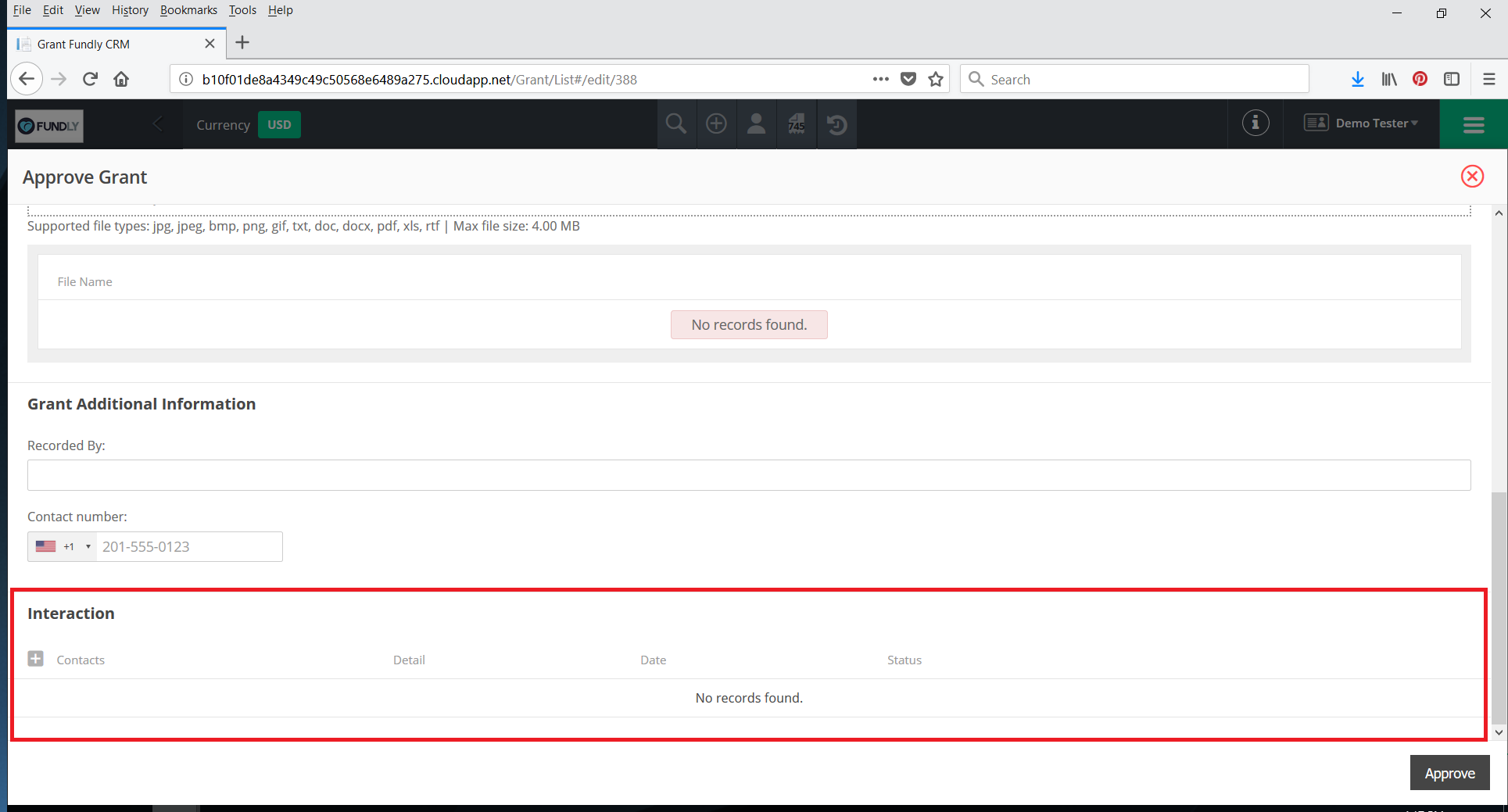The image depicts a rectangular screenshot of a browser window with a gray navigation bar at the top extending from left to right. The gray banner includes traditional menu options on the top left corner: File, Edit, View, History, Bookmarks, Tools, and Help. On the top right corner, there are icons for minimizing, maximizing, and closing the window. One tab is open, labeled "Grant Fundly CRM," with an option to close it.

Below the gray banner, the standard browser interface elements are visible: back and forward arrows, refresh and home buttons, a URL bar, an empty search box, a download icon, and a hamburger menu icon. Directly below this, a black banner spans the width of the window, containing several hard-to-read icons such as a person icon and a search icon, as well as a green box with another hamburger menu. 

In the main content area of the browser, a white box with a white background is displayed prominently with the heading "Approve Grant." It specifies the supported file types for upload: JPG, JPEG, BMP, PNG, GIF, TEXT, DOC, DOCX, PDF, and XLS. There is an upload area for files. At the bottom of this section, a pink box with black text reads "No records found."